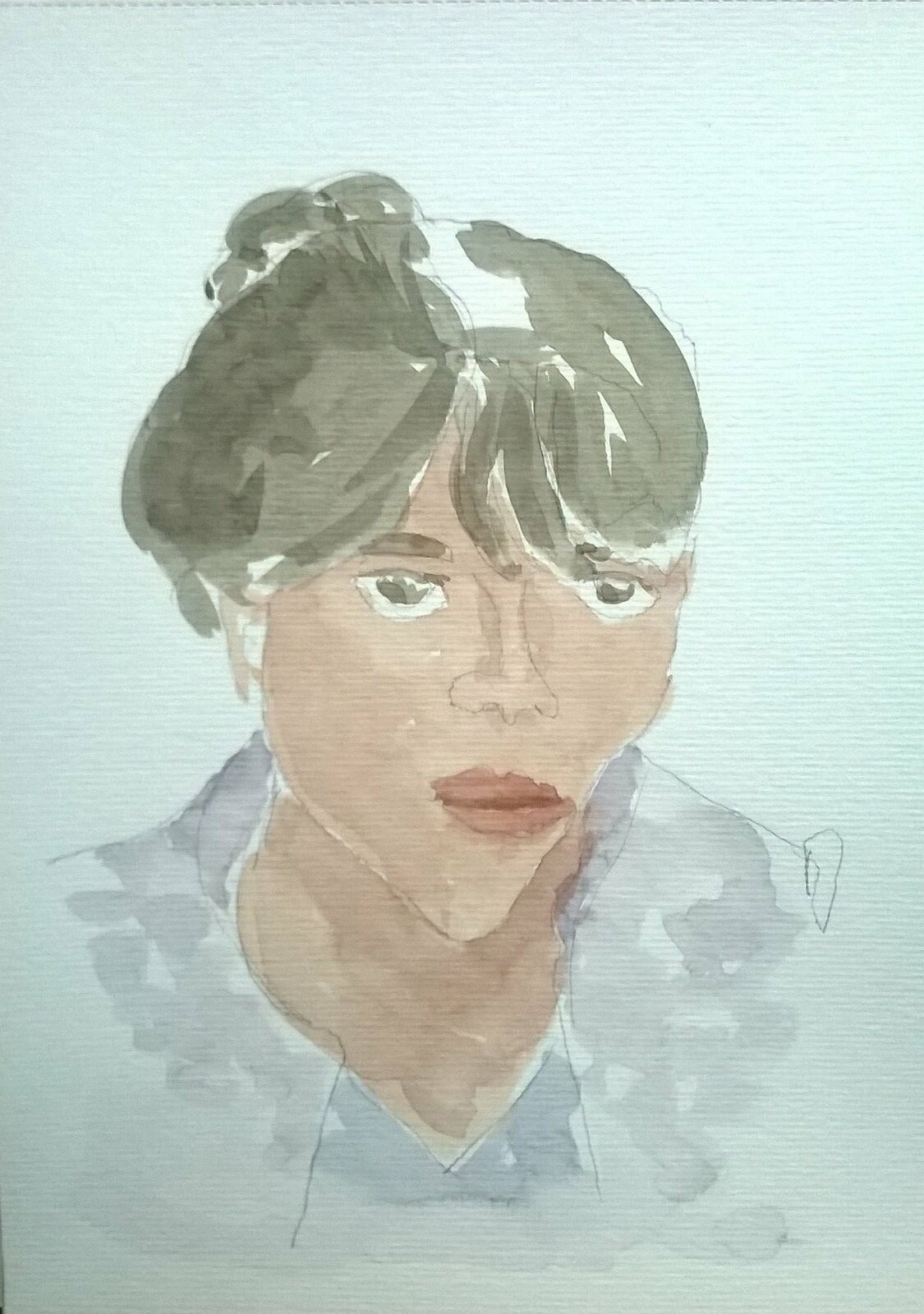This is a light watercolor painting of a Caucasian woman depicted with an impressionistic style on light blue, textured paper. Her hair, appearing in shades of gray and light brown, is pulled back into a bun with bangs nearly reaching her eyes. She features large brown eyebrows, almond-shaped brown eyes, and a petite, slightly misshapen, cone-shaped chin. Her wide lips are accentuated with red lipstick against her pale skin. She wears a v-neck blouse with splotches of blue and white, adding depth to the composition. The portrait's minimal background emphasizes the rough texture of the canvas and the delicate rendering of the figure's face and torso. The expression on her face appears neutral, with eyes gazing forward.